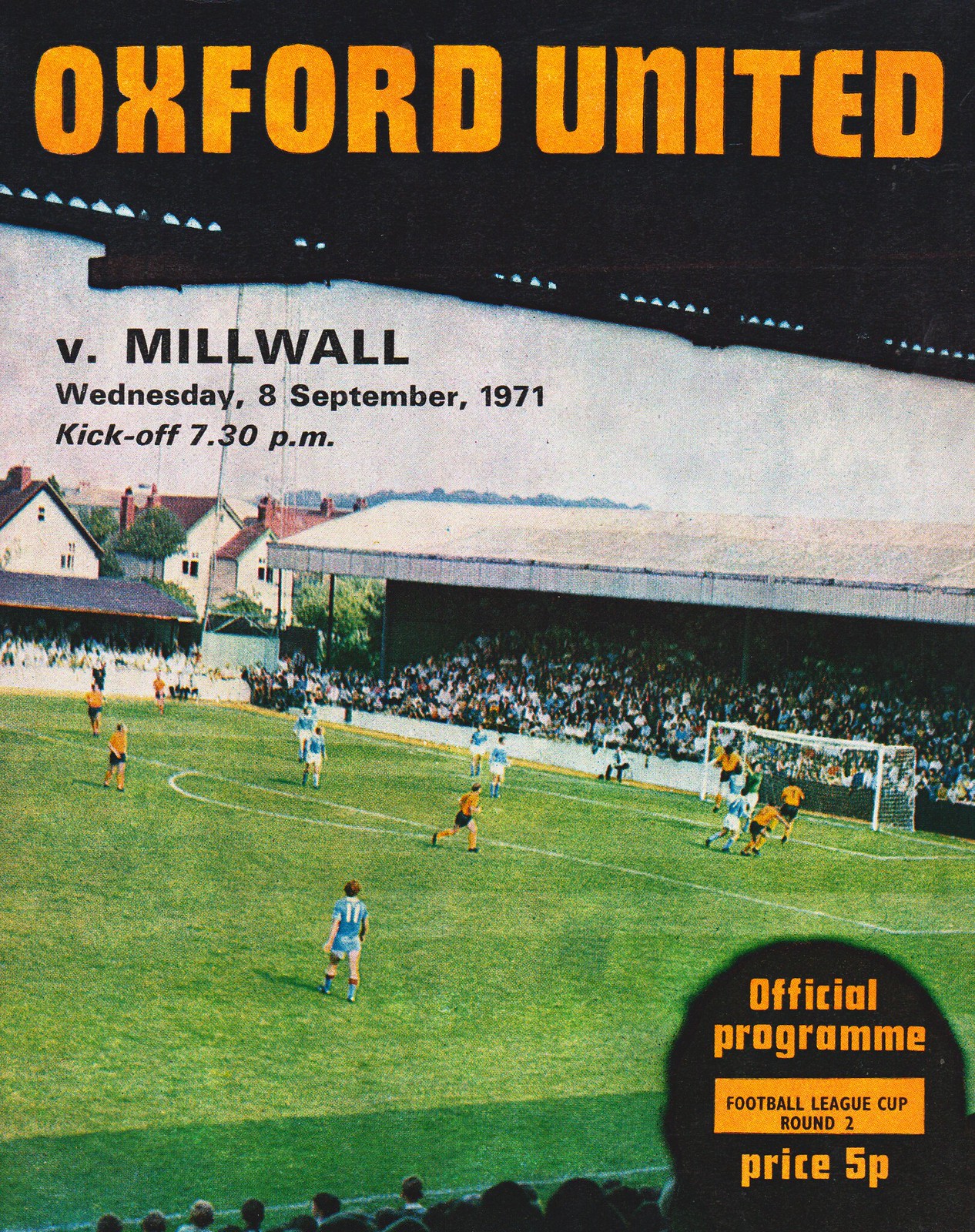This image is a detailed depiction of a soccer program from a match between Oxford United and Millwall on Wednesday, 8th September 1971, with a kickoff time of 7:30 p.m. The top of the program features a black banner with "Oxford United" in bold orange letters, followed by the description "V. Millwall" in black lettering. Below this text, an illustration captures a vibrant live-action shot of a soccer match. The green field is marked with white lines and features a goalpost. The stands, holding numerous seated fans, are situated behind the goal and covered with a white awning. The two teams are distinguishable by their colors: Oxford United's players wear orange jerseys with black shorts and socks, while Millwall's players are outfitted in light blue jerseys and shorts, complemented by blue socks and shoes. The background includes trees, houses, and a clear sky. In the bottom right corner, there is a black circle with orange lettering stating, "Official Program, Football League Cup, Round 2, Price 5p." The scene suggests the match is outdoor and taking place during the daytime, capturing the competitive spirit of the game in a well-detailed illustration.